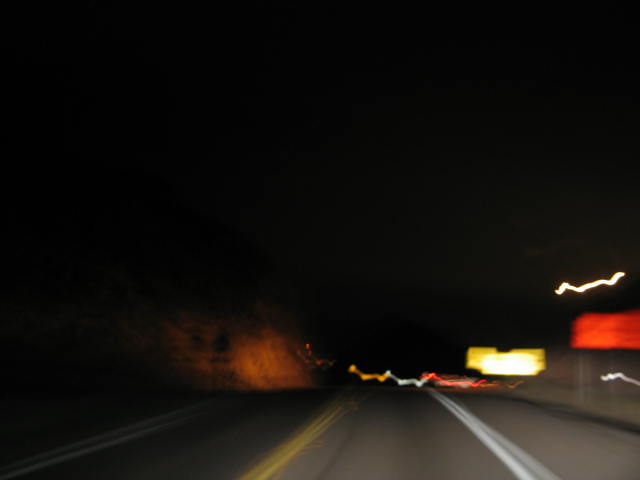This nighttime photograph is taken from what appears to be the perspective of a vehicle traveling down a two-lane highway. The image is heavily blurred due to motion, making it difficult to discern specific details. The road is gray concrete, divided by a yellow center line, with white stripes marking the edges of the lanes. The top half of the image is almost pitch black, characteristic of the night sky. To the right side of the road, you can make out the blurred forms of two street signs, one red and one yellow, possibly indicating advertisements. Ahead on the road, there are blurred tail lights of a vehicle, giving an impression of movement. Additionally, streaks of white light are visible across the scene, further conveying the sense of speed and motion in this dark, out-of-focus shot.